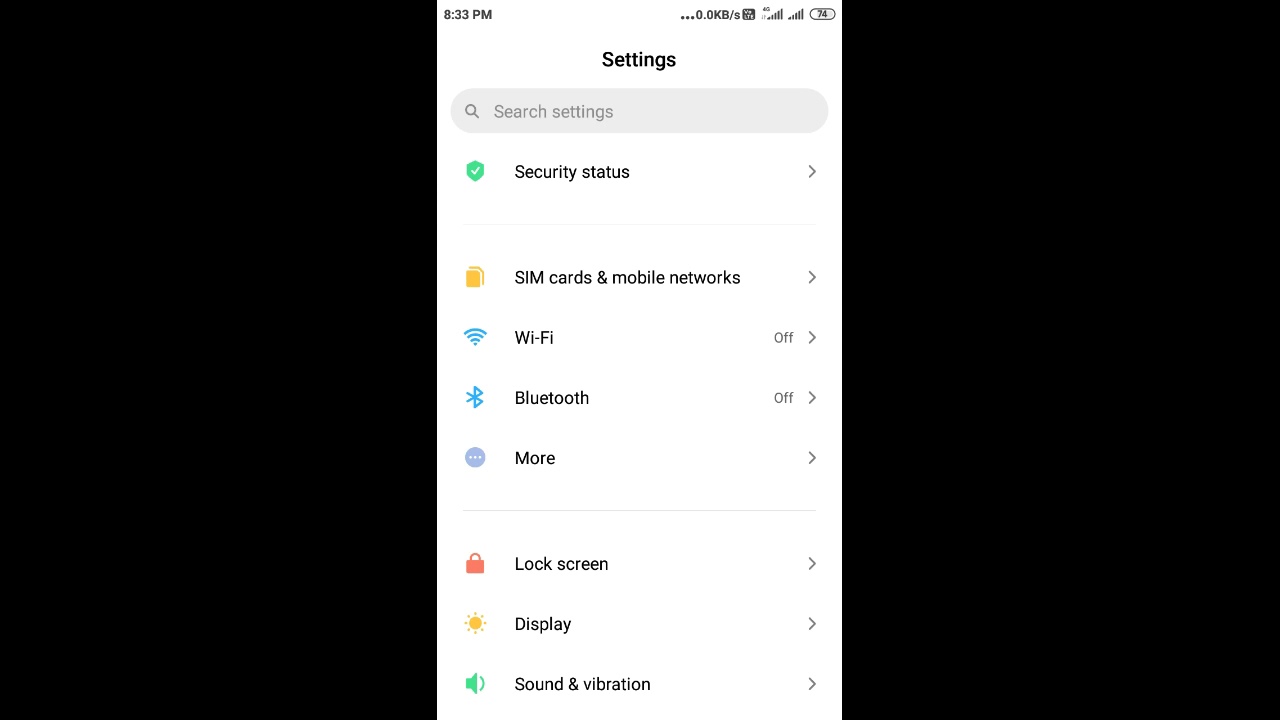This screenshot captures an Android device interface. The screen is bordered by large black bars on both sides, significantly contrasting with the image itself. At the top left, the device time is displayed as 8:33 p.m. To the top right, indicators show two SIM icons and network signals, with the first SIM connected to 4G and Voice over LTE (VoLTE) enabled. The battery is at 74% capacity. The visible text on the screen suggests the user is in the settings menu, listing options such as "Search Settings," "Security Status," "SIM Cards & Mobile Networks," "Wi-Fi," "Bluetooth," "More," "Lock Screen," "Display," and "Sound & Vibration."